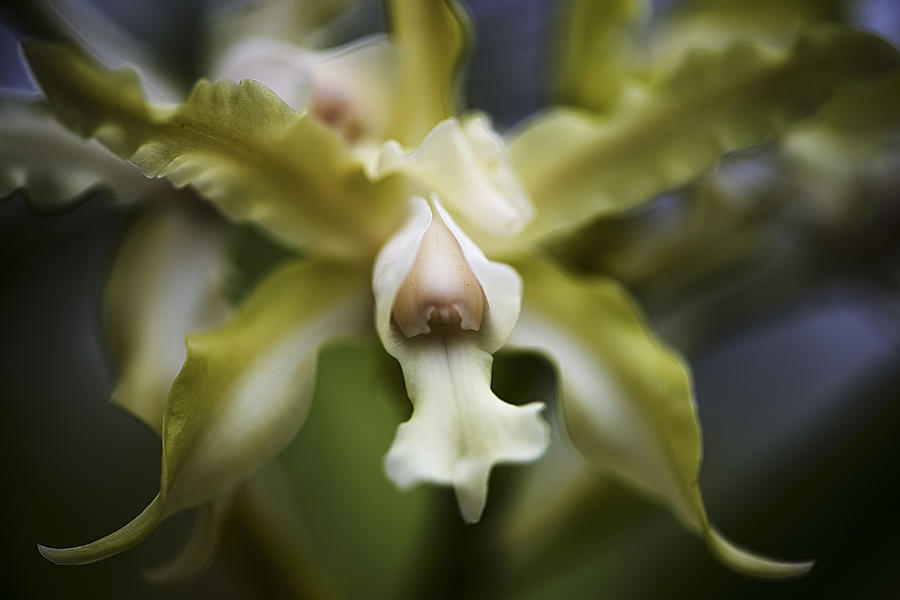This image showcases a close-up of a rare and exotic tropical orchid in full bloom. The flower features four long, slender, ruffled petals arranged in an X shape, with a predominantly yellow hue accented by shades of green. The two upper petals appear darker, while the two lower petals have green outer edges and white inner portions, giving them a crimped texture. Centrally, a striking white stem stretches upwards, flanked by small white petals, leading to a tan, bud-like structure that almost resembles a peeled peanut. The background is dark and blurred, allowing faint glimpses of green leaves and other similar flowers, creating a dreamy, otherworldly ambiance that highlights the intricate details of the orchid.